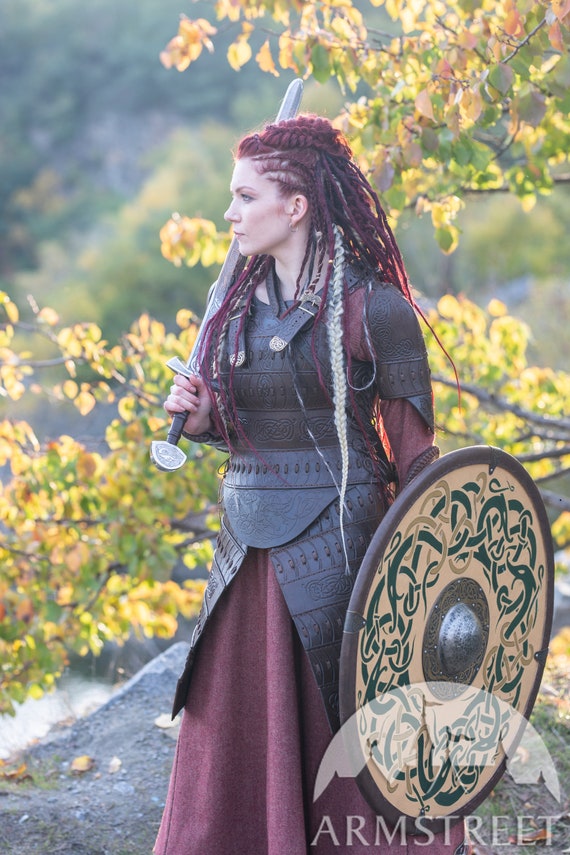In a powerful, muted portrait featuring a woman dressed in elaborate Renaissance or Viking-inspired attire, a white woman with pale skin and striking red braids that descend to her hip stands as the focal point. Her hair includes black and a blonde streak, intricately styled into cornrows or box braids. Clad in a combination of dark brown or silver leather armor and a burgundy dress, she exudes strength and mystique. She holds a great sword in her right hand, resting it on her shoulder, while her left hand grips a large, round shield adorned with a silver center and dark brown edges. The shield's intricate design features interwoven green and gold snake or dragon-like patterns. She stands in an outdoor setting, likely on a hill or cliff, with a sunlit backdrop of blurred green trees, contributing to the image's serene yet powerful atmosphere. In the bottom right-hand corner of the image, a watermark reads "Armstreet," accompanied by a logo resembling a white half-circle with an etched tassel.